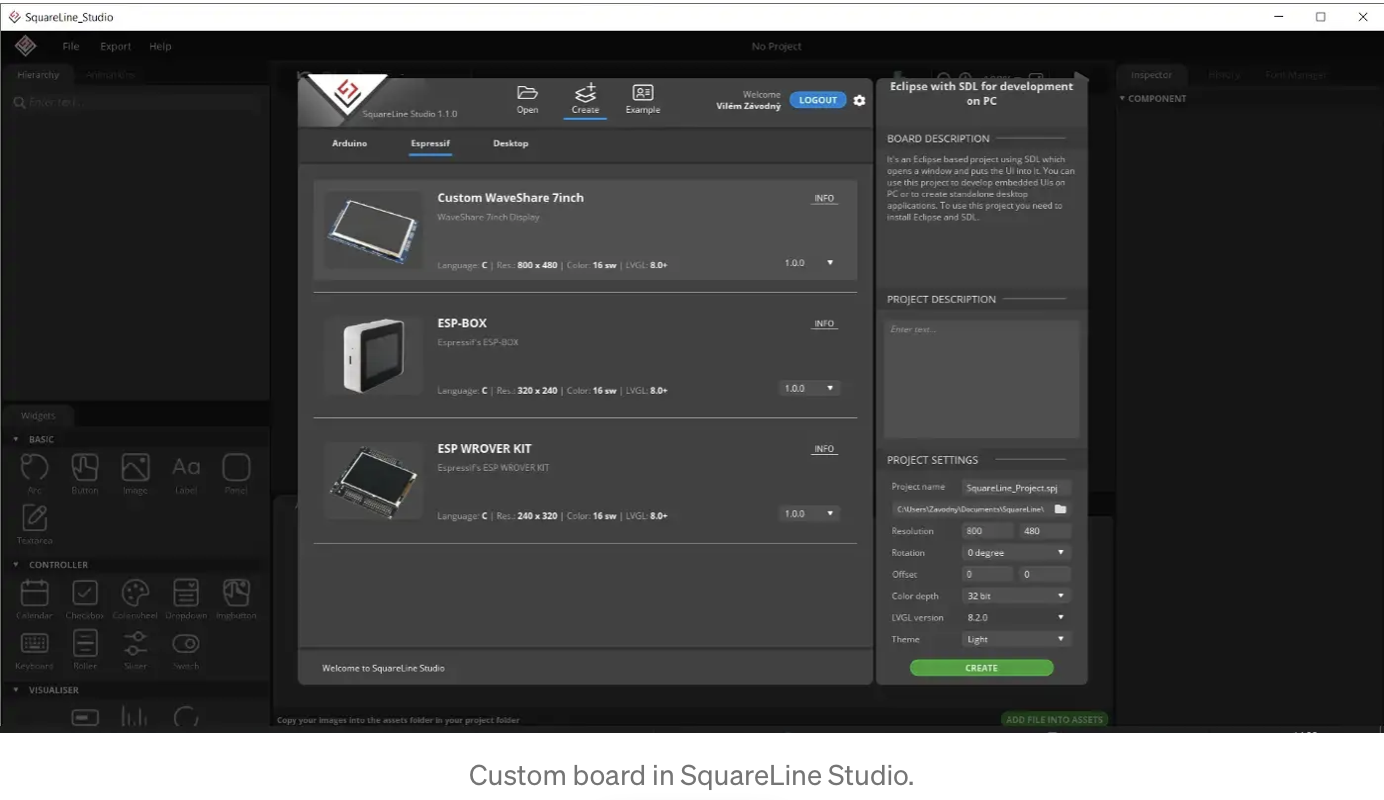The image showcases a sleek website interface with a predominantly black background accented by lighter gray overlays and vibrant blue and green highlights. On the left-hand side, several dialog boxes or widgets are organized vertically, each featuring white icons with labels such as "arc," "button," "image," "label," "panel," "text area," "calendar," "check box," "color wheel," "drop down," "image button," "keyboard," "roller," "slider," and "switch."

In the upper left corner, there are three tabs labeled in white text: "File," "Export," and "Help." At the center of the interface, a lighter gray square overlay prominently displays three featured items. The first item, a digital display, is bolded in white text as "Custom Waveshare 7 inch display." Below this, another digital display is labeled "ESP Box." The third item, a mechanical component possibly resembling a motherboard, is labeled "ESP Rover Kit" in bold white text.

On the far right of this central overlay, detailed text explains the project's context: "Eclipse with SDL for development on PC, followed by more text that reads board description. It's an Eclipse-based project using SDL, which opens a window and puts the UI into it. You can use this project to develop embedded UIs on PC or to create standalone desktop applications. To use this project you need to install Eclipse and SDL."

At the bottom of this central overlay, a series of labeled menus are visible, titled "Project Name," "Resolution," "Rotation," "Offset," "Color Depth," "LVGL Version," and "Theme." Prominently featured below these menus is an oval-shaped bright green button with white text that reads "Create."